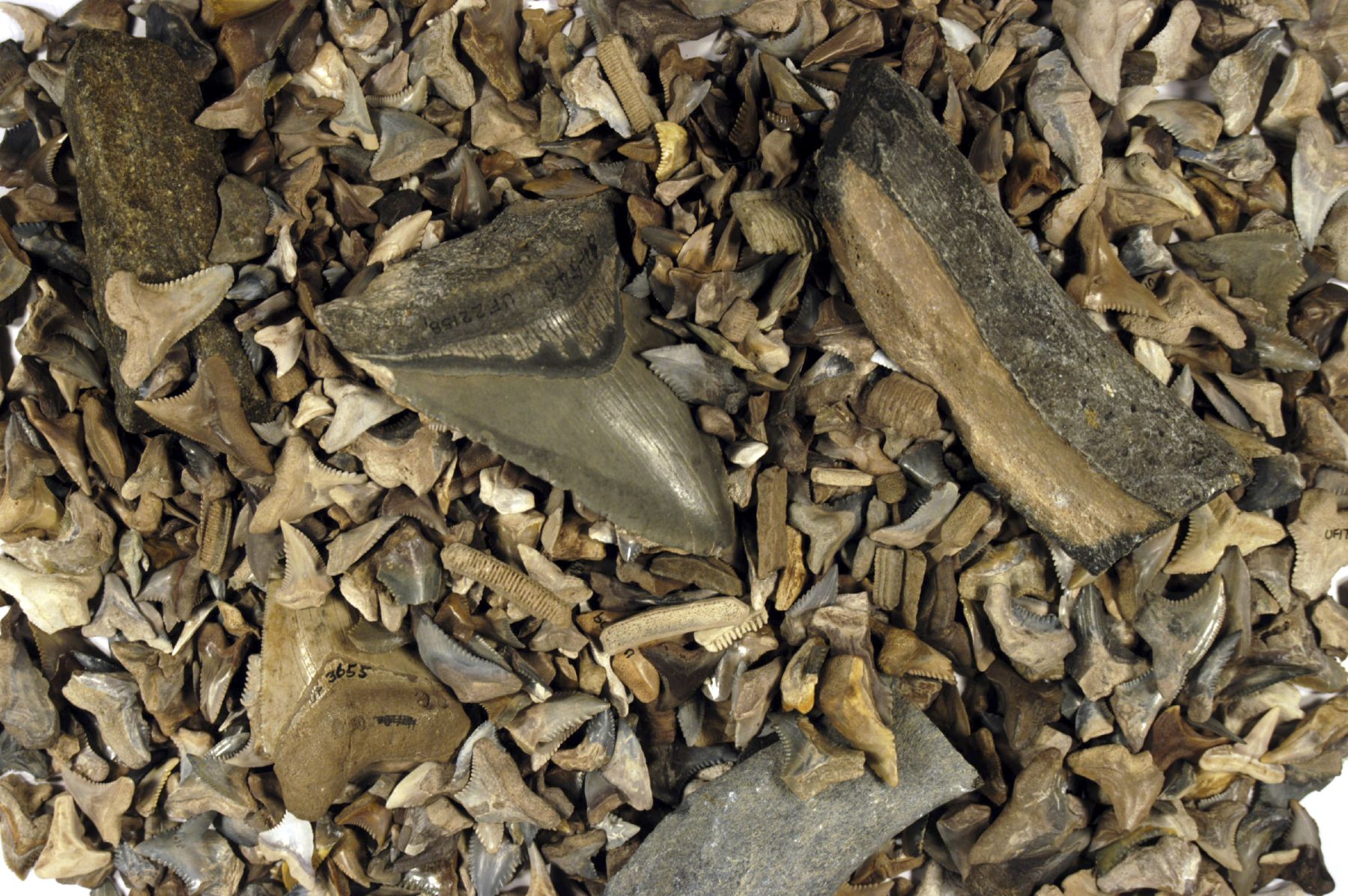This close-up image depicts a top-down view of a surface covered with a large collection of fossilized shark teeth, set against a background of various shades of brown. Among the multitude of teeth, which vary greatly in size and shape, one dominant tooth in the center stands out due to its dark brown color and upside-down triangular form. There are also smaller, miniature teeth scattered around it, many of which exhibit distinct ridged lines characteristic of shark teeth, though some are smooth, elongated, and rectangular, with one light beige tooth noticeable at the tip of the larger tooth. Additionally, the image includes identifiable fossil teeth, such as UF-22158 and UF-3655, marked and cataloged by the University of Florida, emphasizing the scientific significance of the collection. Fragments that might resemble bones, pebbles, or pieces of wood add to the intricate detail seen across the composition.